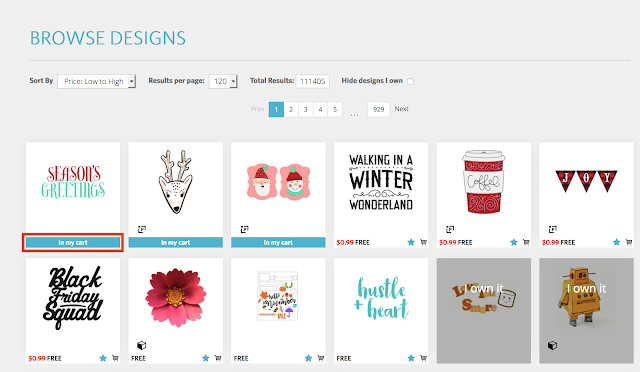In this image, we observe a screenshot of a website presented against a very light gray background. In the upper left corner, large blue text displays the website's name, "Browse Designs." Below this heading, there is a sort options box, displaying "Price: Low to High" with a pull-down menu for further sorting preferences. To the right of the sort box, the text "Results per page: 120" specifies how many items are shown per page. Further to the right, there is an option labeled "Hide designs I own" accompanied by a small checkbox. The screen also indicates the total number of pages available, revealing 929 pages, with the first page highlighted in blue.

The main section of the screenshot showcases a gallery of colorful images arranged from left to right. The first image in the gallery shows a white box with the phrase "Season's Greetings" written on it, followed by an image of a reindeer head. Next to it, there are two snowman-like characters. Further to the right, in black text, the phrase "Walking in a Winter Wonderland" is visible. 

On the second row, in the lower left position, there is text in cursive that reads "Black Friday Squad", and next to it, to the right, another box contains a pink flower.